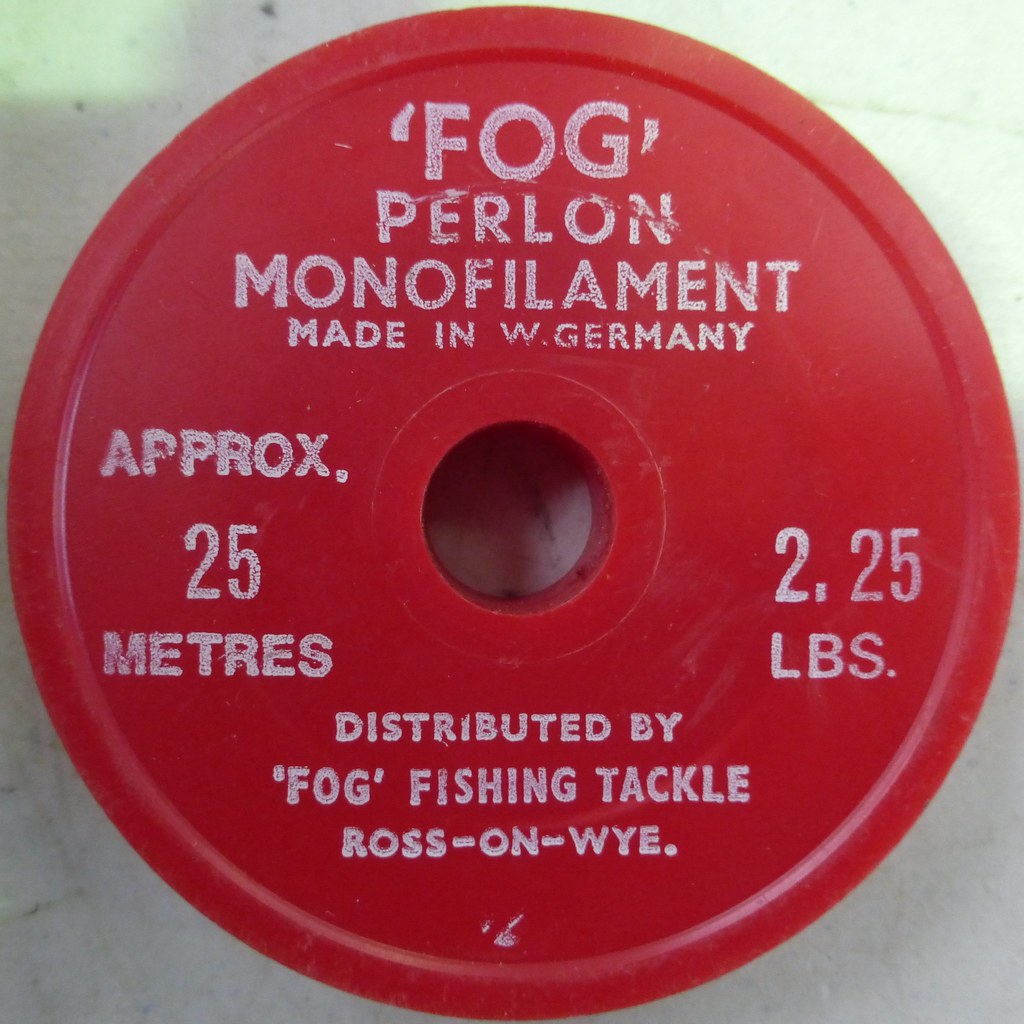The image shows a round red plastic object, resembling a spool, resting on a white table with yellow and dark streaks. The object appears to be about 8 to 10 inches in diameter and features a central hole approximately two inches wide. Inscribed in white letters on the red plastic are the words "Fog Perlon Monofilament," and below that in smaller text, "Made in West Germany." To the left is the phrase "approximately 25 meters," and to the right, "2.25 pounds." At the bottom, it says "Distributed by Fog Fishing Tackle, Ross-on-Wye." The design and inscriptions suggest it is related to fishing tackle, possibly used for holding or dispensing fishing line.